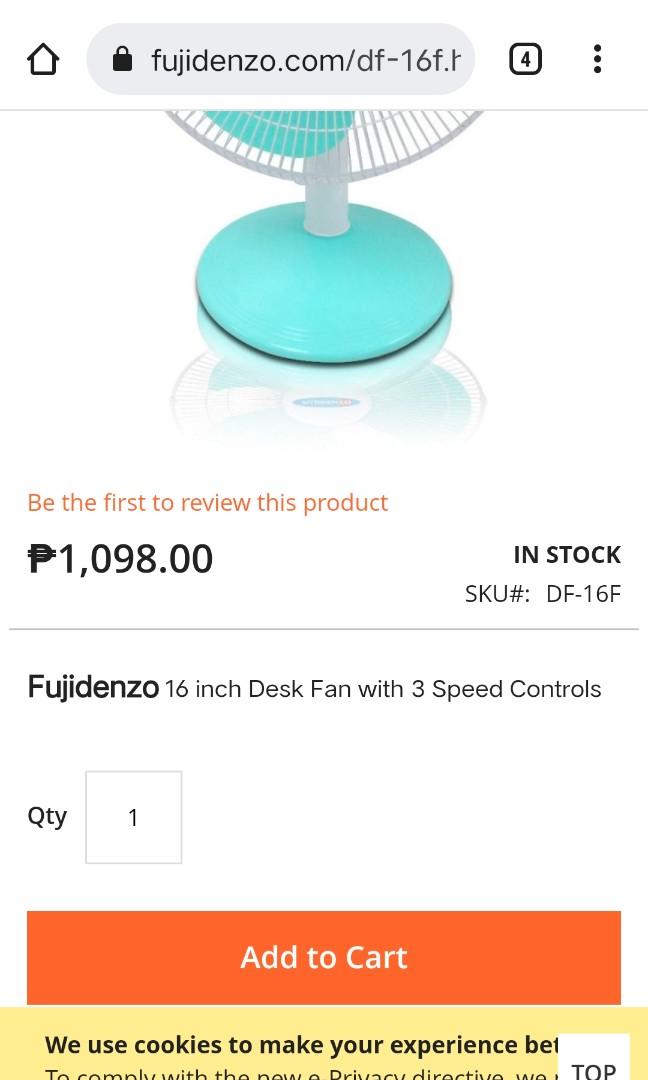**Detailed Caption:**

This is a vertical screenshot of a website, fujidenzo.com, viewed on a smartphone. The interface indicates the mobile browser environment with options to navigate home on the top left and three circles on the top right, suggesting additional settings. The browser tab section shows that four tabs are currently open.

The website's background is predominantly white. The URL is prominently displayed at the top center. Below it, a partially visible image of a mint green fan with white hardware appears, hinting at the product being showcased. Below this image, an orange text reads, "Be the first to review this product," indicating that there are no existing reviews.

The price of the fan is listed as 1,098 Philippine pesos, with an "In Stock" status highlighted in bold black font. The SKU number is provided as DF-16F. The product name, elaborately titled "Fujidenzo 16 inch desk fan with three speed controls," is clearly visible below the SKU.

Further down, there is an option to adjust the quantity, currently set at one, adjacent to an orange "Add to Cart" button with white text. At the very bottom of the screen, a yellow box with black text partially reads, "We use cookies to make your experience bet," with the remaining part of the word "better" cut off by a white box labeled "Top," designed for quick navigation to the top of the page.